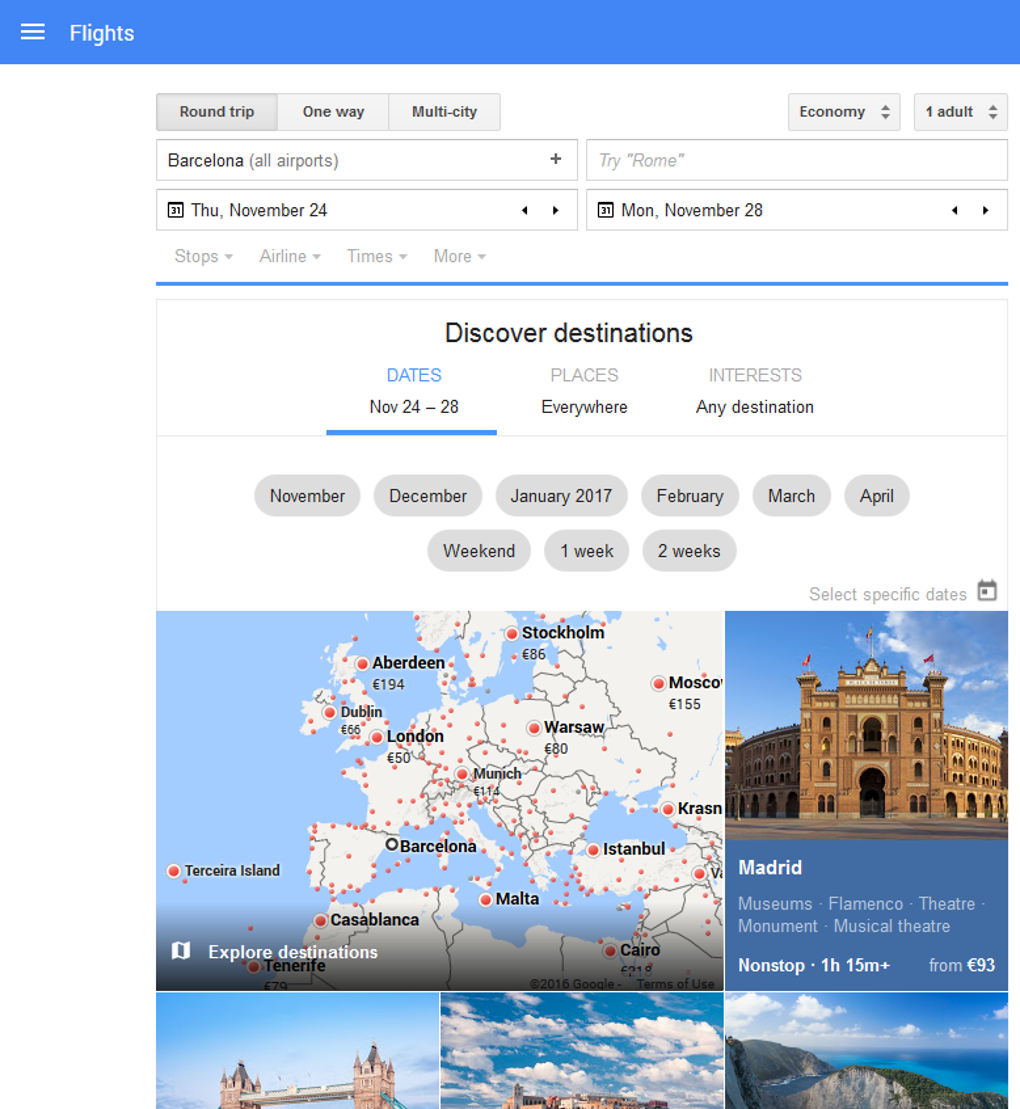The image presents a flight booking page, characterized by its detailed layout and a comprehensive array of options. In the top left corner, various flight choices are visible, including "Round Trip," "One Way," and "Multi-City," alongside booking classes like "Economy." The page specifies details for one adult traveling from Barcelona (All Airports) on a round trip scheduled from Thursday, November 24th to Monday, November 28th.

The interface includes a menu icon and gives the user the ability to discover destinations. Date options displayed span from November through April, with suggestions for various trip durations—weekend getaways, one-week, and two-week vacations. An interactive map highlights potential destinations, including Aberdeen, Stockholm, Warsaw, Moscow, London, Munich, Barcelona, Saqqara (Ireland), Casablanca, Malta, Istanbul, Cairo, and Madrid.

Flight reminders such as a non-stop flight that lasts 1 hour and 15 minutes from €93 are also noted. Additional images and locations are sprinkled throughout the page, along with associated flight fees to provide comprehensive travel options to the user.